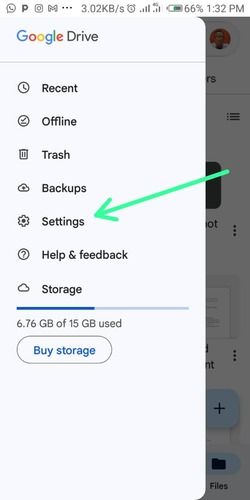Screenshot of a Smartphone Interface with Google Drive Menu Open

The screenshot captures a smartphone interface with various notification icons at the top, indicating active phone alerts, a 'P' notification, a camera icon, data rate of 3.02 KB/s, a clock icon, signal bars, and battery life at 66%. The time displayed is 1:32 p.m. 

The main focus of the screenshot is the Google Drive application, currently open and covering most of the screen. The Google Drive header is prominently displayed at the top, with "Google" in its signature multi-colored letters and "Drive" in black text. 

Beneath the header is a series of menu options in a neatly organized list. They include:
1. **Recent**, indicated by a clock icon.
2. **Offline**, marked with a check in a circle.
3. **Trash**, accompanied by a trash can icon.
4. **Backups**, featuring a cloud symbol.
5. **Settings**, denoted by a cogwheel icon, which is highlighted by a green arrow pointing towards it.
6. **Help and Feedback**, represented by a question mark in a circle.
7. **Storage**, also accompanied by a cloud icon.

Under the list, a storage usage bar is displayed. It is predominantly light blue with a dark blue section indicating the used portion. The storage statistics reveal that 6.76 GB of the available 15 GB has been utilized. The storage bar is clickable, offering further interaction.

The background of the phone screen is minimally visible due to the overlay of the Google Drive menu, providing a focused view on the application's interface and options.